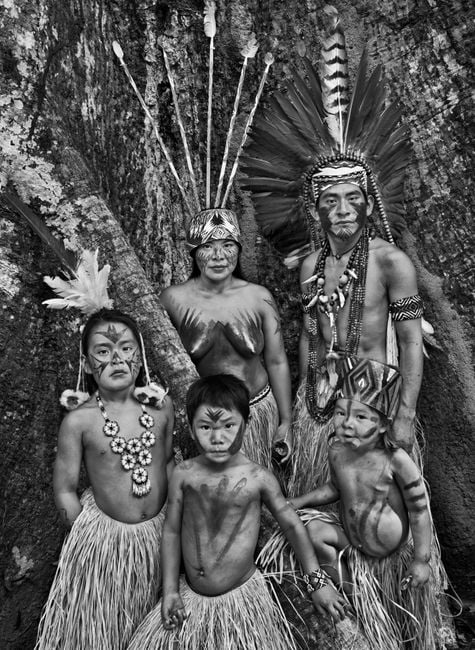The photograph captures an indigenous family of five, likely from Southeast Asia or the South Sea islands, standing before a majestic oak tree. The family, consisting of a father, mother, and three children approximately aged 10, 8, and 6, are adorned in traditional attire. All members are dressed in grass skirts and are shirtless, showcasing their intricate body paint and jewelry. 

The father is distinguished by his large, feathered headpiece, several necklaces, likely made from animal teeth, and dark splotches of paint on his cheeks. The mother, in the background, has her chest artistically painted and wears a headdress with pipe-like structures and five arrows sticking out. 

The children in the foreground display varied body paint patterns: one child features a V-shaped design on their chest, another has three dark stripes on their shoulder, and the third has a whisker-like design and a diamond pattern on their forehead. One child wears an ornate, tall hat with an interlocking diamond pattern design and necklaces, while another has a feathered headpiece and an armband. This detailed depiction emphasizes their cultural heritage and the intricate beauty of their traditional regalia.